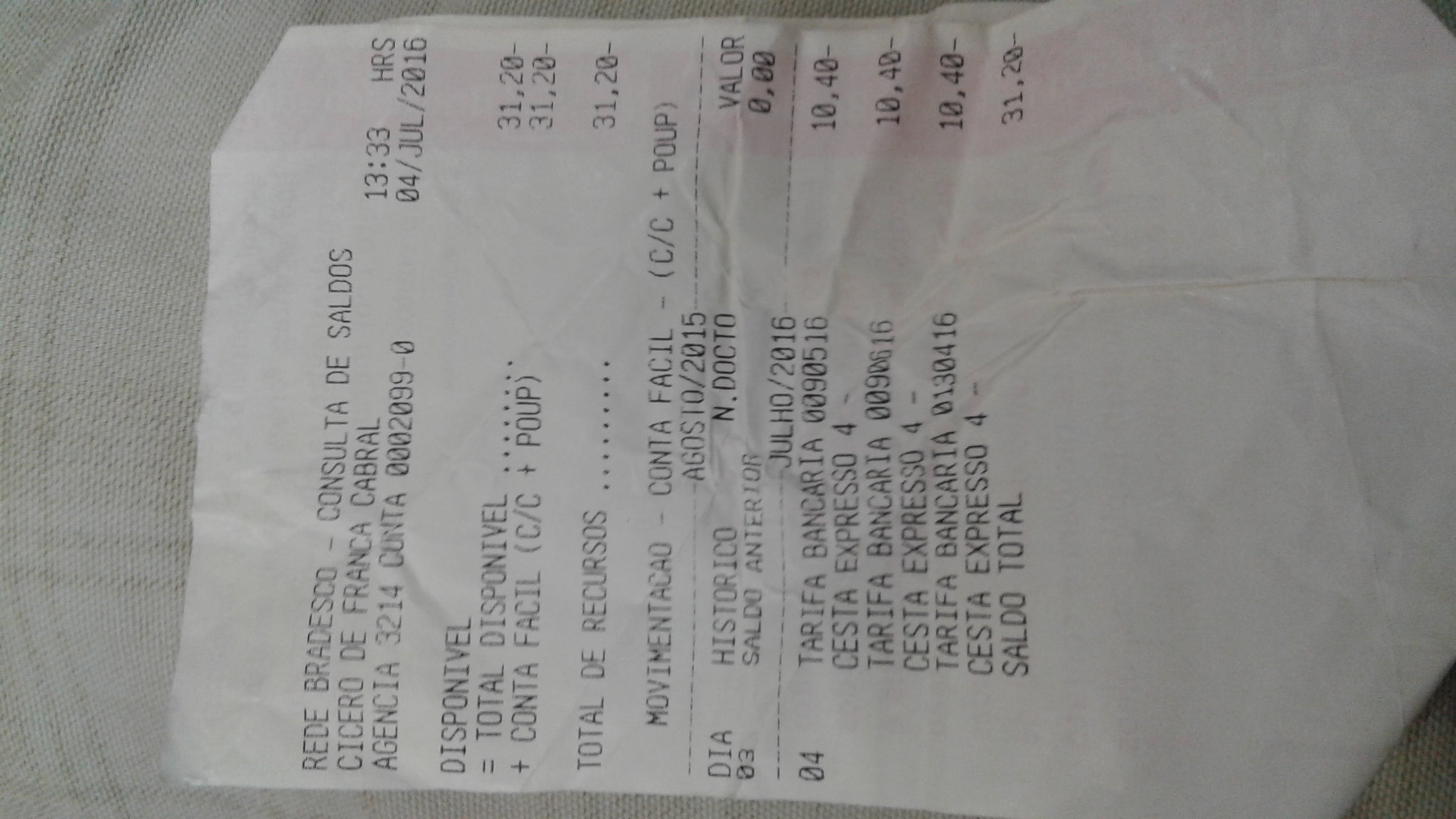A crinkled and folded receipt lies sideways on a white and gray striped woven cloth, giving it a textured appearance. The receipt, dated July 4, 2016, at 13:33 hours, is primarily in Spanish and suggests it was issued by Bradesco, a bank or finance-related institution. It details the purchase of three coffees, each priced at £10.40, making a total of £31.20. The receipt also includes various banking terms like "historial," "saldo," "tarifa bancaria," and mentions a bank fee or tax. The overall appearance of the receipt, combined with the bilingual text, hints at an international context, possibly a transaction involving multiple currencies.